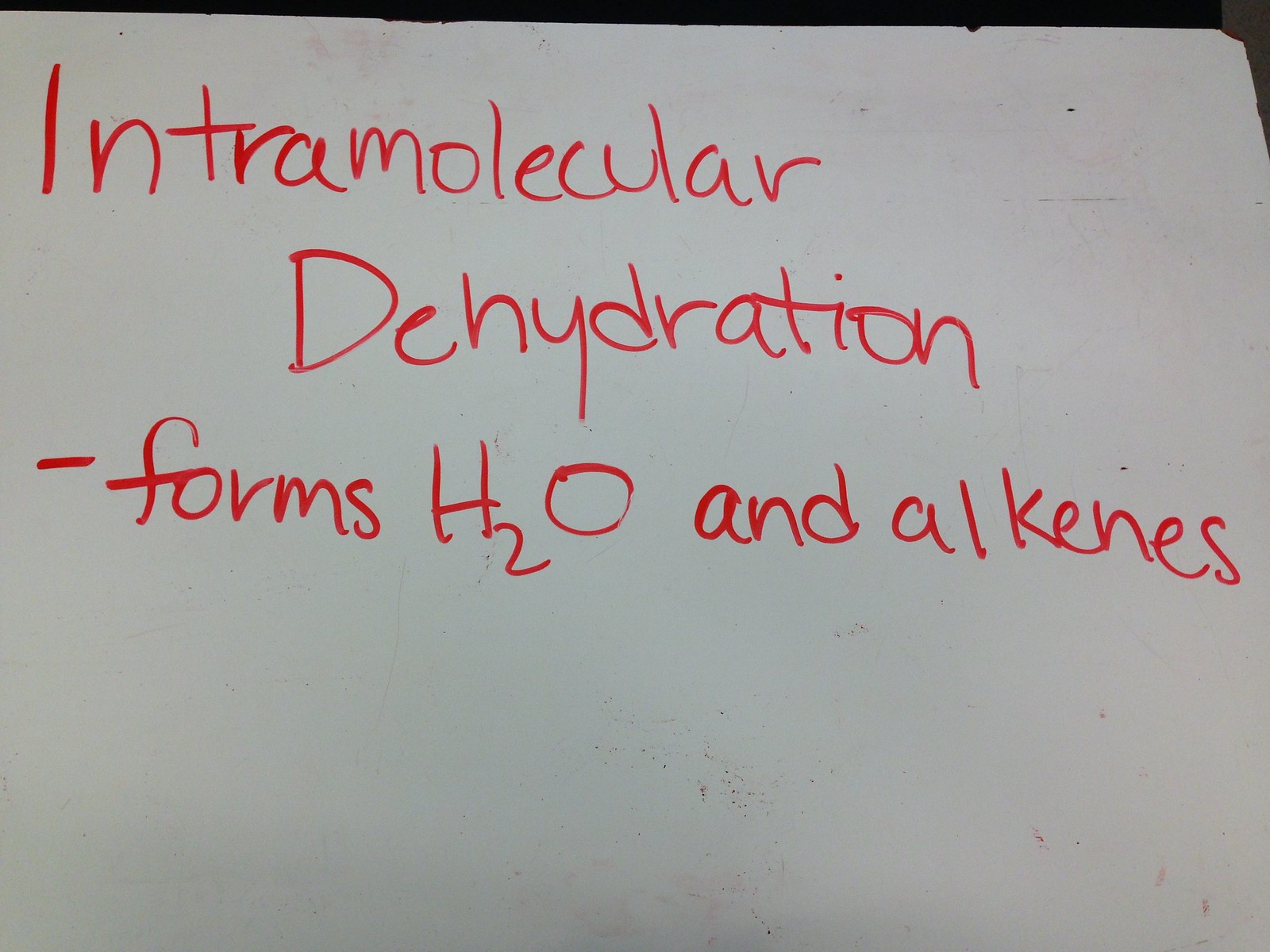The photograph captures a well-used, somewhat dirty whiteboard, displaying signs of wear, including smudges, specks, and previous erasing marks. The top right corner of the board is distinctly visible, appearing black due to shadows and the angle of the photograph. The whiteboard is inscribed in red marker with three lines of text occupying the top two-thirds of the surface. The handwriting, although legible, is not particularly neat. The first line reads "Intramolecular," the second line reads "Dehydration," and the third line reads "— Forms H2O and Alkenes." The lower one-third of the whiteboard is blank and marked with various remnants of old writings and erasures, giving the board an overall worn and beat-up appearance.